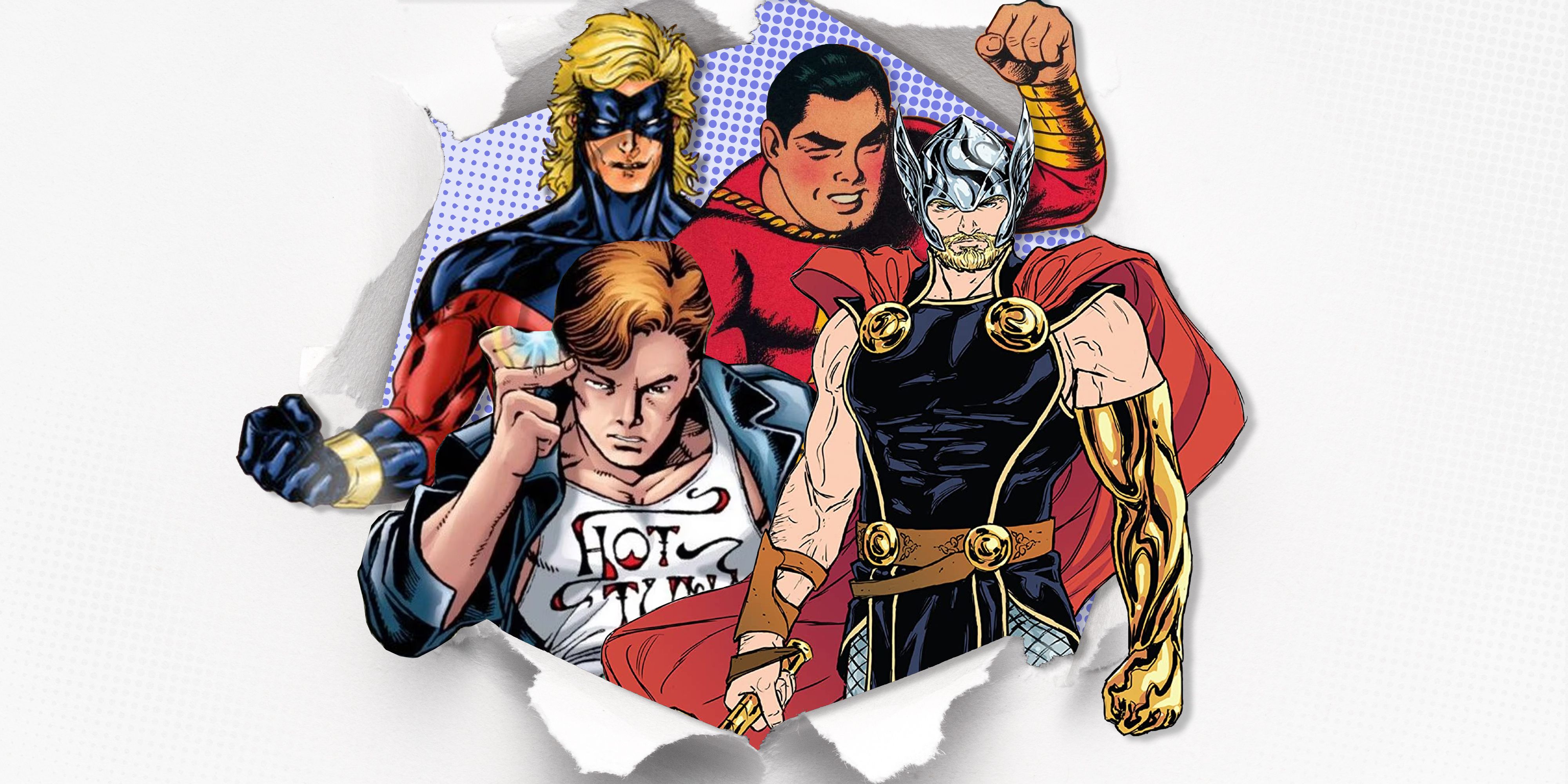In the center of this image, a large circular tear in white paper reveals a dynamic scene featuring several classic comic book heroes. Prominently displayed in the foreground is Thor, distinguished by his silver winged helmet and black, sleeveless costume adorned with four large gold buttons. He wears a red cape with gold trim, and his left arm is encased in a gold glove extending to his bicep, while his right hand holds an undefined object. To the left, Shazam stands out in his vintage 1950s appearance, donning a red costume with a gold rope fastened around his neck and a matching red cape. Behind Thor, a muscular figure deep in thought presses his hand to his temple, while another hero with yellow hair and a blue mask stands nearby. Completing the ensemble is a man in a yellow uniform with a cape and gold wristbands. These characters appear to burst through the paper, evoking the vivid and nostalgic art style of 1980s comic books.